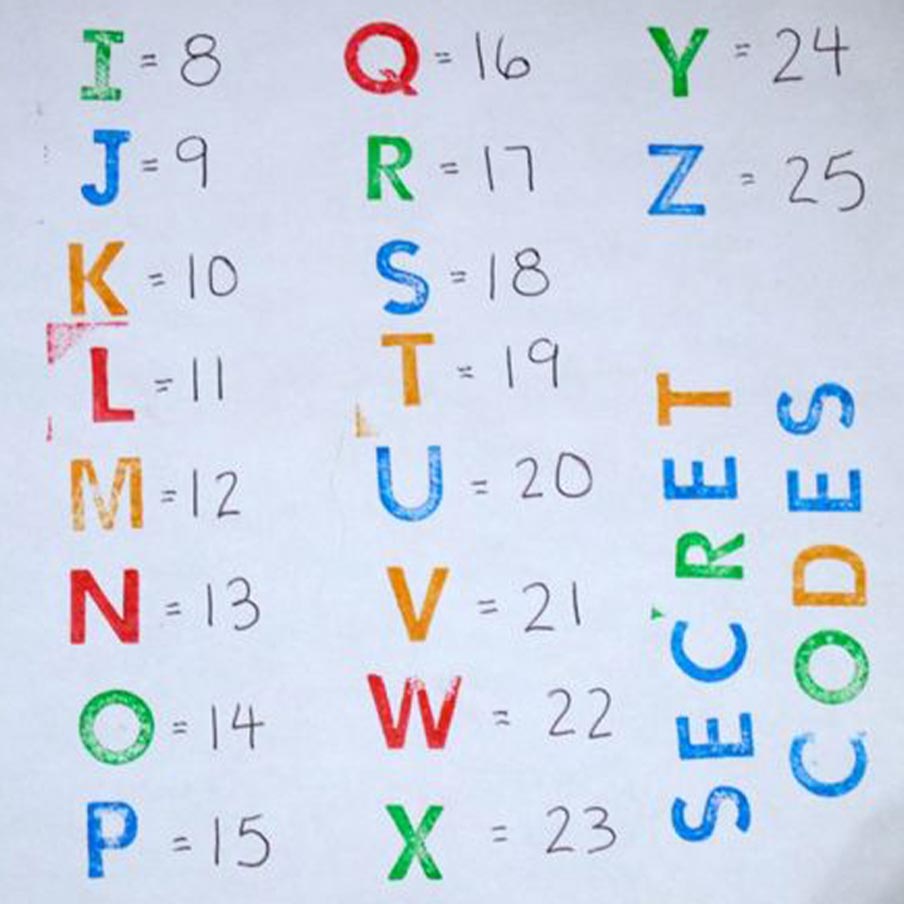This image showcases a chart titled "SECRET CODES" in the bottom right-hand corner, written vertically so that you would need to rotate the paper to read it correctly. The chart features capital letters I through Z, each paired with a corresponding number ranging from 8 to 25. The elements are presented in three columns against a white background. Each letter is boldly colored in green, blue, orange, or red. Specifically, the pairings are as follows: I (green) equals 8, J (blue) equals 9, K (orange) equals 10, L (red) equals 11, M (orange) equals 12, N (red) equals 13, O (green) equals 14, P (blue) equals 15, Q (red) equals 16, R (green) equals 17, S (blue) equals 18, T (orange) equals 19, U (blue) equals 20, V (orange) equals 21, W (red) equals 22, X (green) equals 23, Y (green) equals 24, and Z (blue) equals 25. The equal signs and numbers are all handwritten in black, adding a personal touch to the chart's clean, organized presentation.